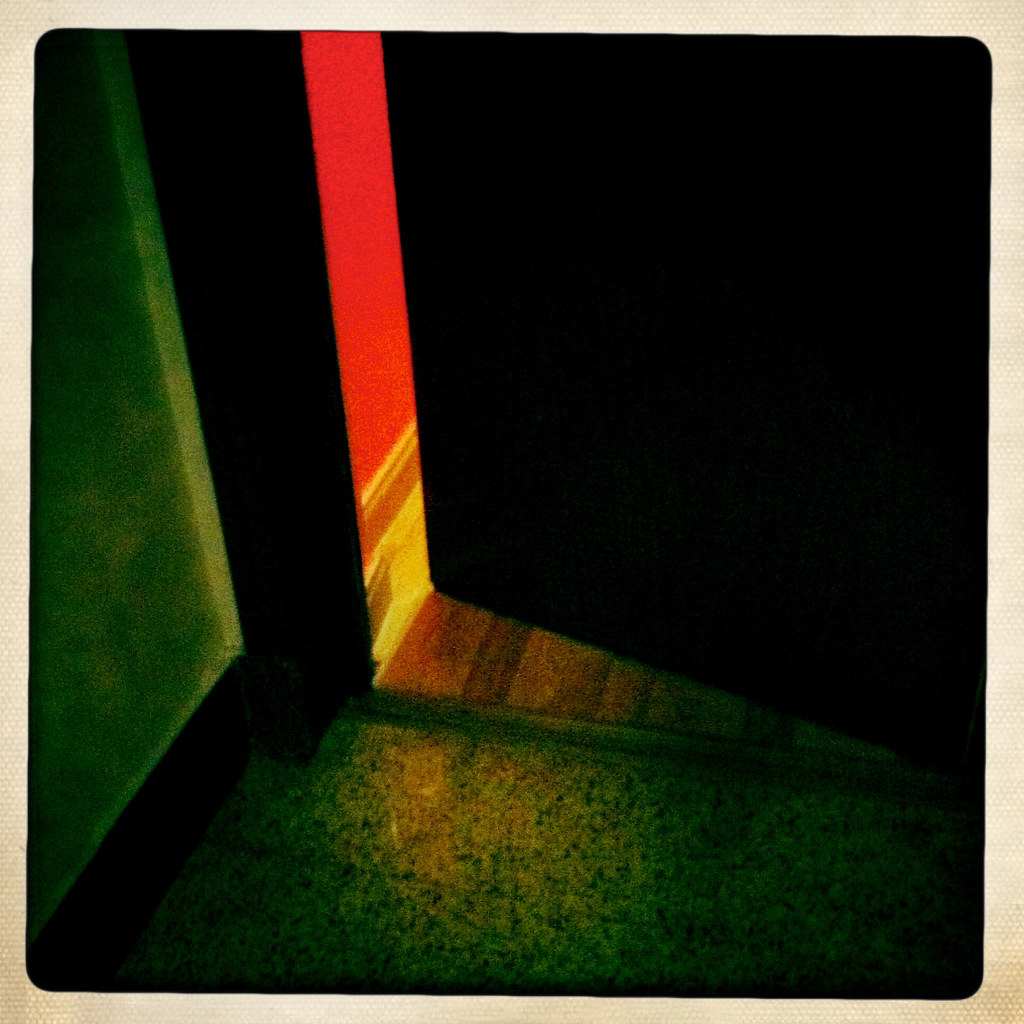The image is a large, square, and very grainy photo that could also be a drawing, depicting a partially opened black door. The bottom of the image features speckled gray and black tiles transitioning to brown tiles and then to wood flooring as you move upward. On the right side, there is a white baseboard against a red wall, while on the left, a green wall with black baseboards and doorframe is visible. The door is slightly ajar, revealing a room illuminated by a bright light, contrasting with the dimly lit overall setting of the image. The bright light from inside the room accentuates the red wall with the white baseboard at the bottom. The scene appears to be set inside a home, but no people or text are present in the image.